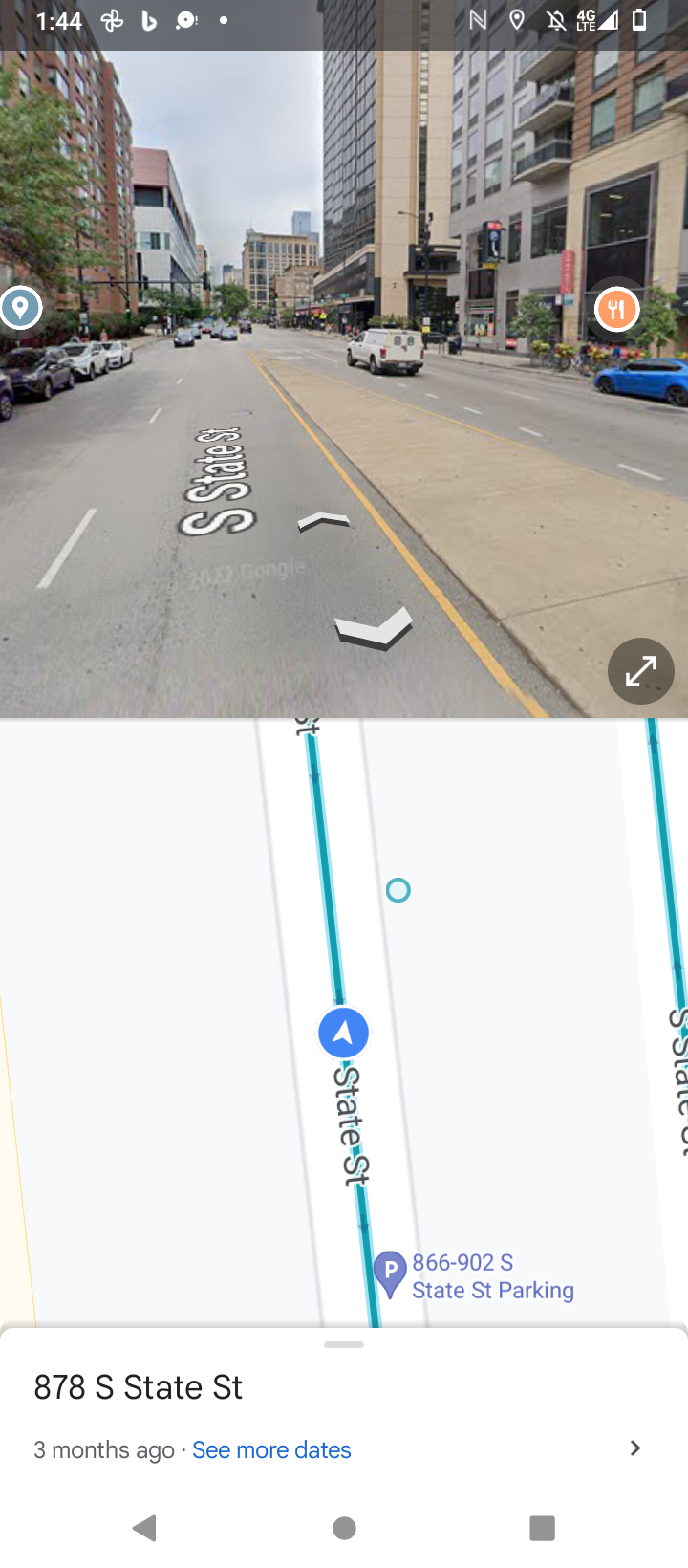**Caption:**   
A screenshot of Google Maps' Street View, captured at 878 South State Street three months ago, features a detailed urban scene. At the bottom, the street is depicted with a distinct blue line and directional blue arrow. The street, named State Street, includes parking spaces as indicated by the "State Street parking" label. The road is marked by a concrete median that divides the southbound and northbound lanes. A blue car is parked on the side of the road, adjacent to an orange circle icon featuring a fork and spoon, likely indicating a nearby restaurant. To the left of this icon, a map marker symbol is visible. Several cars are parallel parked along both sides of the road, and on the right side, the rear of a white utility truck is seen in motion. The image vividly captures the everyday hustle and bustle of this busy street.